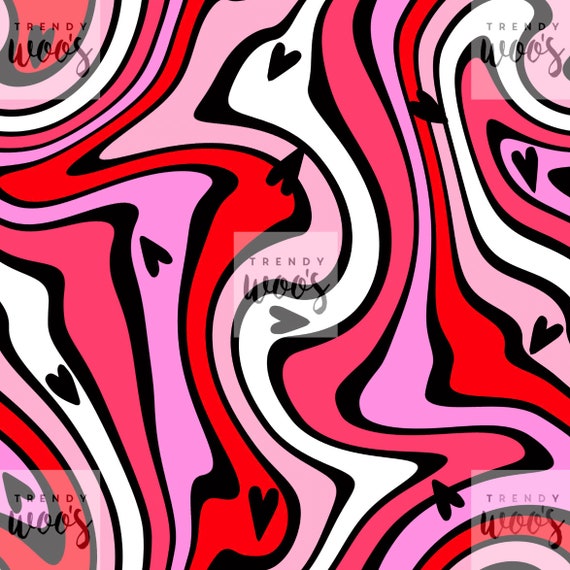This is a vivid and dynamic abstract square graphic, reminiscent of trendy Instagram art. The image is dominated by curvy, squiggly lines in shades of red, pink, white, and purple, outlined in black. These lines and squiggles create a sense of movement, drawing the eye from top to bottom and left to right across the image. Scattered throughout are small, black hearts facing various directions, adding a whimsical touch. The graphic features multiple translucent watermarks that read "Trendy Woos," positioned in each corner and at the center. Some patterns within the squiggles evoke the shapes of body parts, such as legs or elbows, further enhancing its abstract nature.